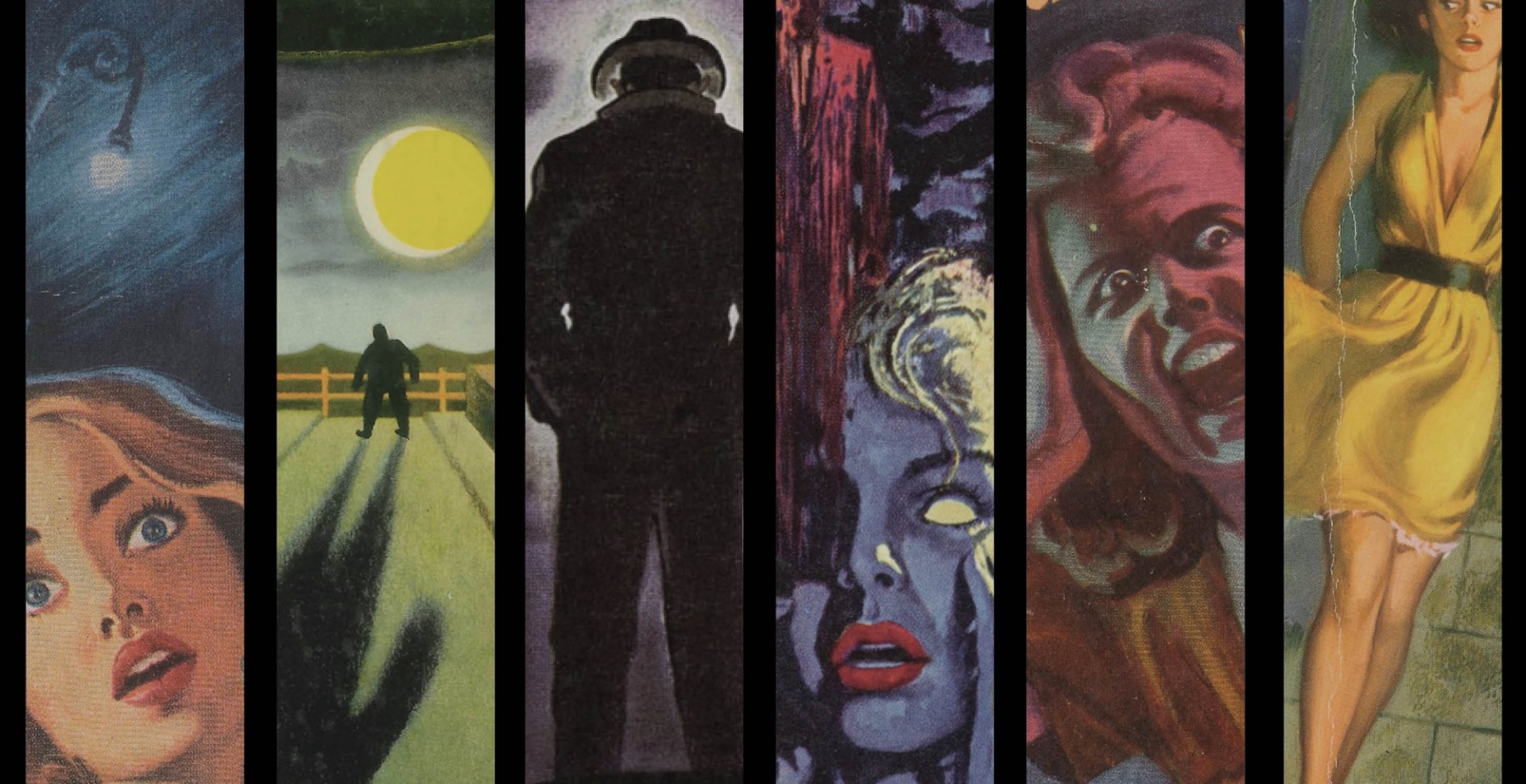The image is a detailed painting divided into six vertical panels, resembling a well-painted, realistic comic strip or storyboard. The panels are much taller than they are wide, even though the overall image is wider than it is tall, creating a unique composition. 

In the first panel, there is a young woman with blonde hair who bears a striking resemblance to actress Margot Robbie. She appears very frightened, with a look of surprise and fear in her eyes, illuminated by a mysterious light. The second and third panels feature a large, shadowy figure that could be seen as menacing; the figure is outdoors as the sun sets, with the back view in one panel showing a possible hero-esque figure wearing a hat.

The fourth to sixth panels return to the young woman, whose expressions portray escalating fear. In these panels, she transitions from fear to terror, and in the final panel, she is seen beginning to run, presumably trying to escape the looming threat depicted in the earlier panels. The cohesive sequence across the panels emphasizes a narrative filled with suspense and urgency.